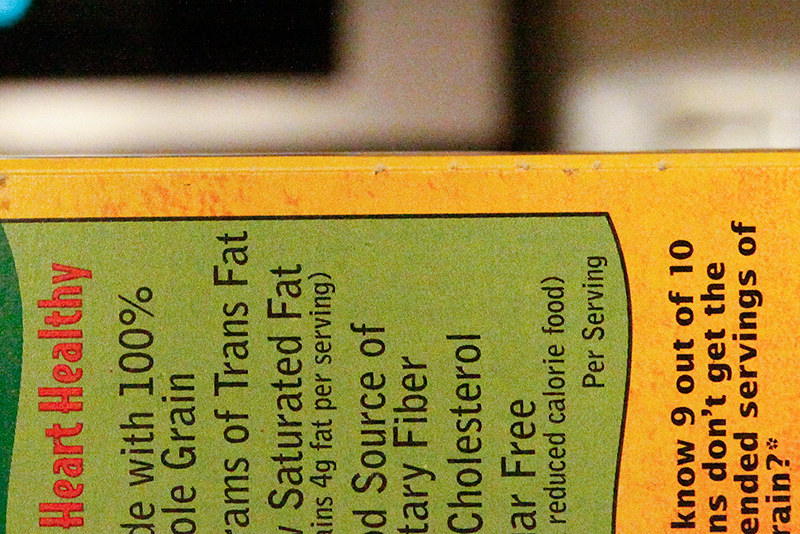The image depicts the back panel of a food product box, which is lying on its side, rotated a quarter turn to the left. The box itself is made of cardboard and is predominantly orange. The back panel features an olive green section bordered in black. At the top of this green section, bold red letters proclaim the product as "Heart Healthy." Although partially visible, the text continues with phrases like "with 100% whole grain," "grams of trans fat," "source of fiber," "cholesterol," "something free," and "reduced calorie food." Below the green panel, on the orange part of the box, additional text is partially legible, stating "no 9 out of 10, something...don't get the something."